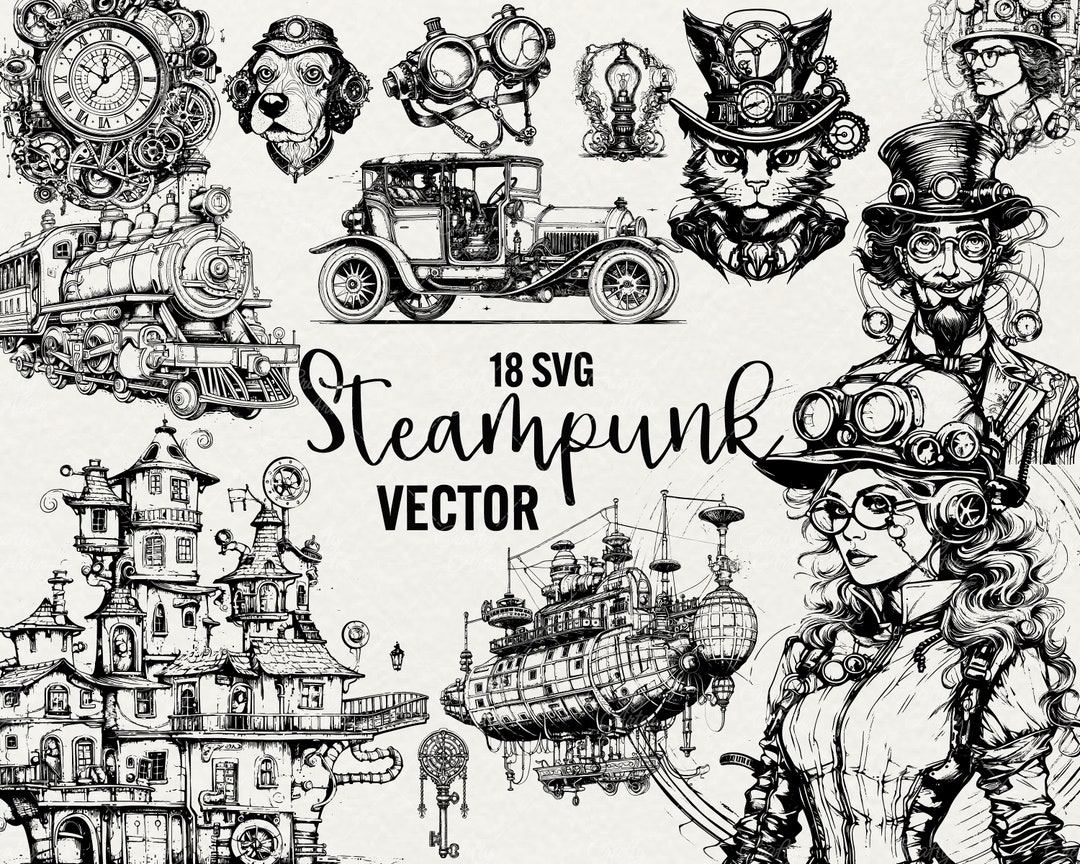This highly detailed black-and-white poster serves as an advertisement for steampunk enthusiasts, prominently featuring the text "18 SVG Steampunk Vector" in its center. Encompassing a variety of intricately drawn steampunk-themed elements, the poster includes images of a man and woman, both wearing distinctive steampunk attire such as goggles, hats, and vintage glasses. Additionally, it depicts various creatures, including a dog and a cat, both adorned in period-appropriate accessories.

Around the central text, the poster showcases elaborate steampunk vehicles and structures: a vintage four-passenger car with an open front and a solid roof, seemingly from the late 1800s or early 1900s, sits near the top of the design. A fantastical airship, resembling a precursor to a blimp with a boat-like structure below it, is laden with small windows, parapets, doohickeys, and an observation deck. Drawn below this are a large ornate key and a highly intricate house, complete with parapets, multiple levels, doors, and windows, resembling a scene from a fantasy world.

Further details include a locomotive engine and an ornately designed clock with visible gears, set to 10 minutes before 12. The entire poster is framed with various steampunk imagery, creating a captivating advertisement for fans of this imaginative genre.